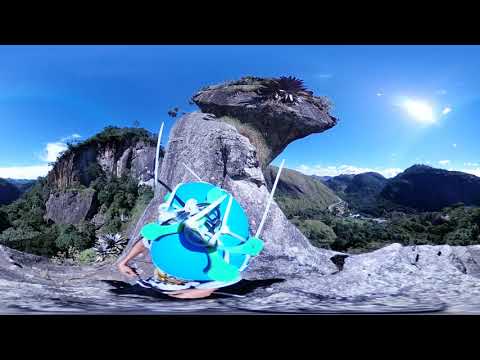The image depicts a tranquil outdoor scene dominated by a prominent, interestingly shaped granite rock face by the water's edge. This granite formation, primarily gray and black, features a top section reminiscent of a dinosaur's or mushroom's head, which has a flatter area with foliage growing on it, creating the illusion of a neck. To the left, we see a large, cliff-like rock face with lush greenery on top, while to the right, mountainous terrain covered with trees and other vegetation stretches into the distance. The scene is bathed in warm sunlight from a blue sky dotted with white clouds. 

In the foreground, a small, circular turquoise raft rests on the shore, which appears to have either been left there or tied up. Additionally, there is an aspect of the image that suggests it might be an advertisement for climbing equipment, as a climbing rope with green and white straps is attached to the raft. This rope could indicate climbing activity, hinting at a climber’s gear setup for spending the night on the mountainside. The overall composition of the image, enhanced with a wide-angle lens, introduces some distortion, emphasizing the rugged beauty of the landscape and the unique granite formation.